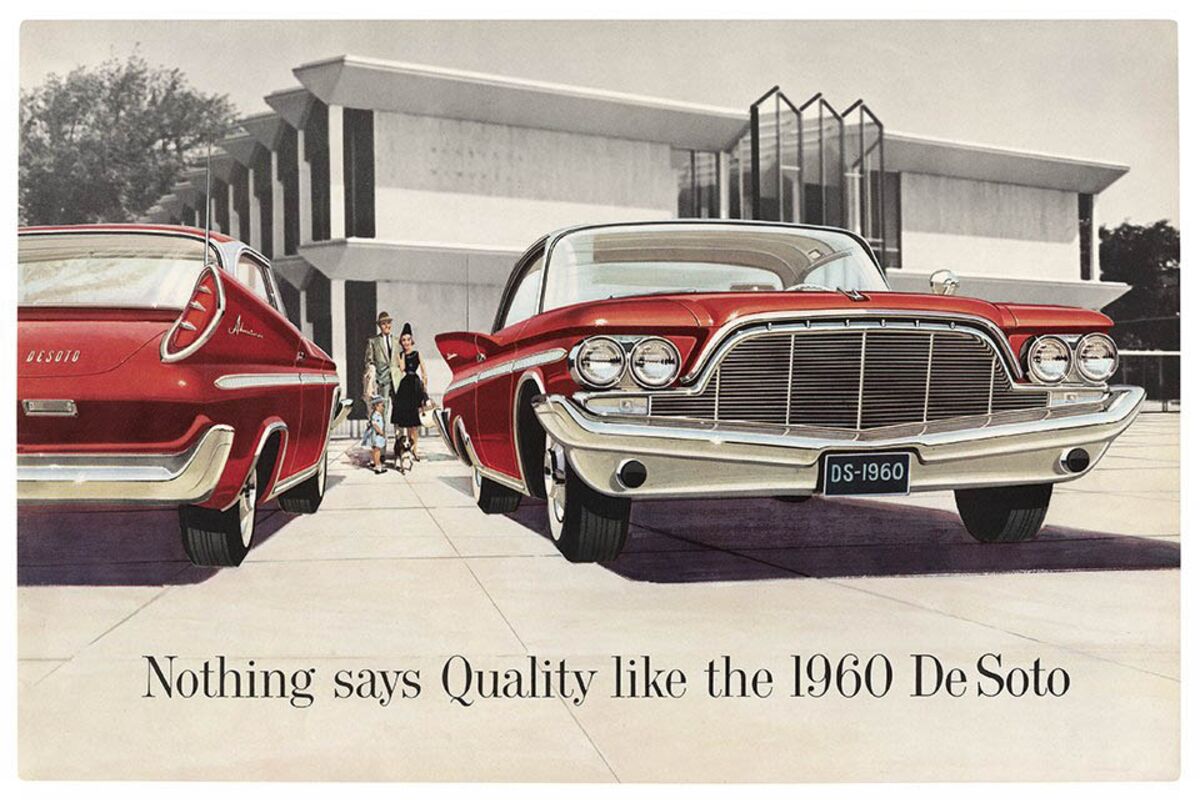The image is an advertisement, predominantly in black, white, and gray tones with vibrant red accents highlighting two 1960 DeSoto cars. The advertisement's tagline reads, "Nothing says quality like the 1960 DeSoto." One car is positioned facing forward, while the other is angled to showcase its distinctive tail fin and taillight. Both cars, in pristine condition with a distinguishing white stripe and white roof, epitomize the classic 1960s style. They are parked in front of a modernistic, space-age home typical of the era, surrounded by trees. A nuclear family consisting of a man, woman, child, and dog is seen walking between the two cars, adding a warm, inviting touch to the scene. The family and the cars are the only colorized elements in what appears to be an intricately detailed drawing. A black license plate on the car to the right reads "DS1960," further emphasizing the model year of these stylish vehicles.